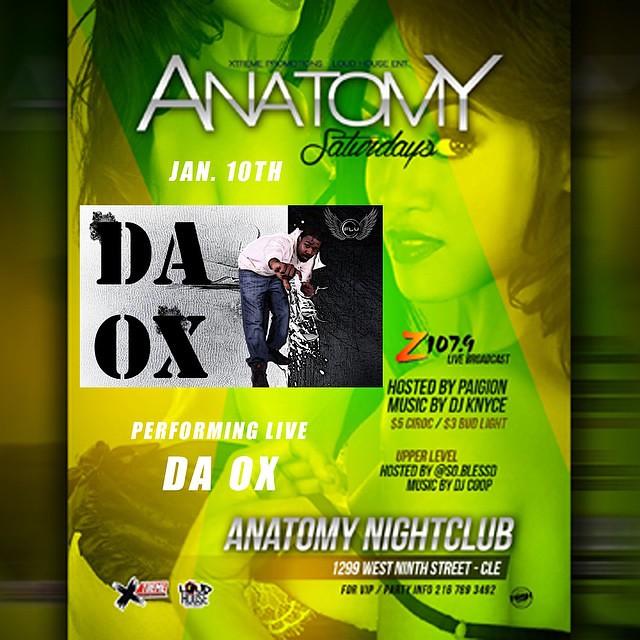The advertisement is vibrant with a green and yellow background, promoting an event titled "Anatomy Saturdays" at Anatomy Nightclub. The event is set for January 10th and features a live performance by the artist DAOX. The central figure in the ad is a man wearing a white sweater, blue jeans, and black shoes, pointing directly at the camera. His name, DAOX, is prominently displayed next to him. Above his image, it mentions the live performance and that the event is hosted by Zia 107.9 with Pajon hosting and DJ Kintz providing the music. The nightclub's address, 1299 West 9th Street in Cleveland, is clearly mentioned. The background subtly includes two faded images of women, one with her face visible looking to the right, and the other with only half her face visible on the left, adding to the visual intrigue. Additional logos are present in the bottom left corner, though they are hard to decipher. The overall design is vertical, making it a striking advertisement for the event.